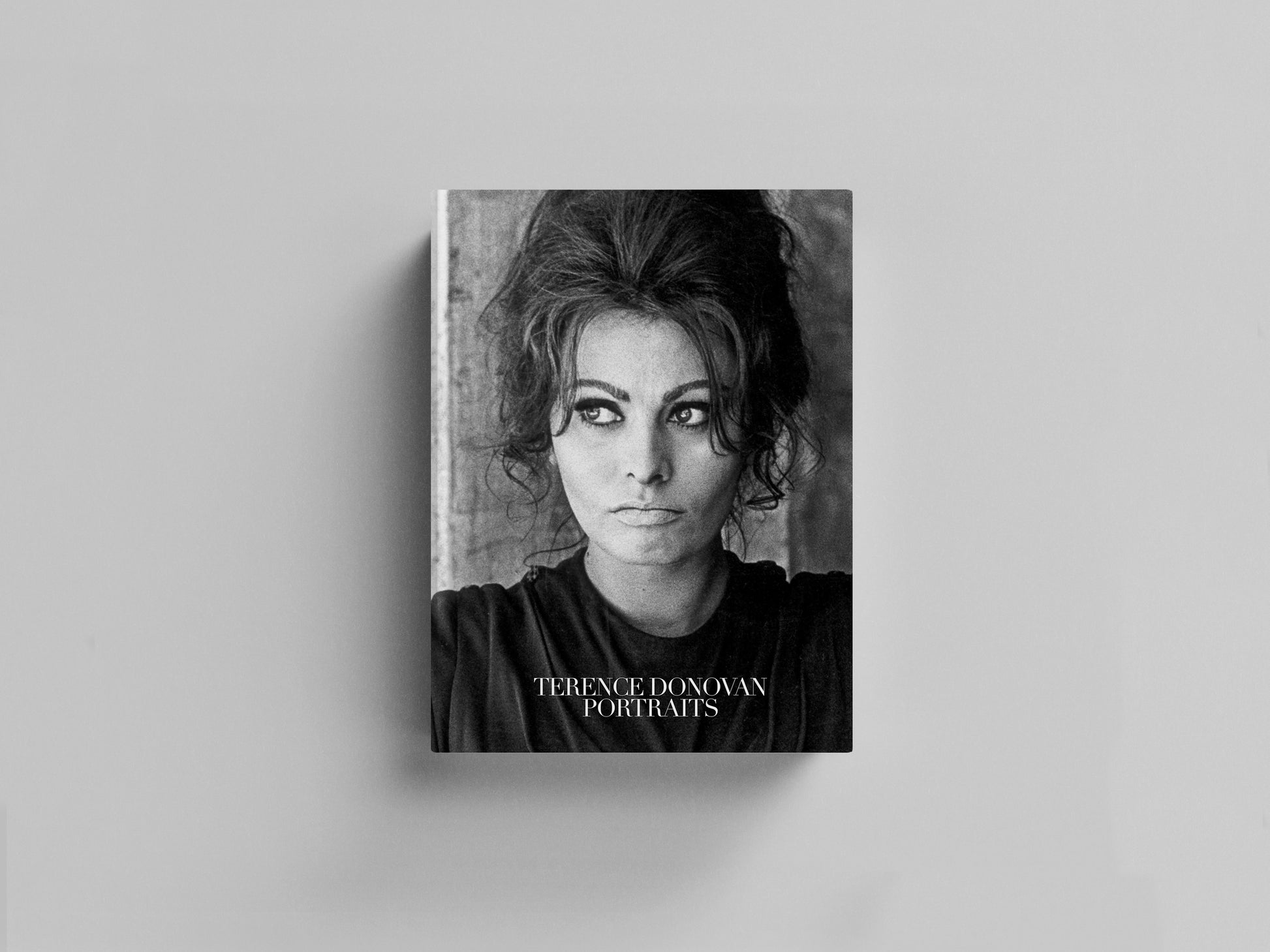The image, presented in black and white tones, reveals a book titled "Terrence Donovan Portraits" prominently centered against a light to medium gray background. The background features various textures and striations ranging from black to brown, suggesting a potentially wooden or textured wall. The book's cover showcases a close-up portrait of the iconic actress Sophia Loren. Sophia is depicted with her hair styled in a messy bun, some strands falling delicately around her face and behind her neck. Her expressive eyes are lined with dark makeup, enhancing her poised gaze directed to her right. She wears an oversized, loose black crewneck shirt, and her expression is neutral, exuding sophistication and calm. The book cover stands upright, casting a subtle drop shadow that adds a sense of depth to the image, reminiscent of professional product photography typically found on e-commerce platforms.